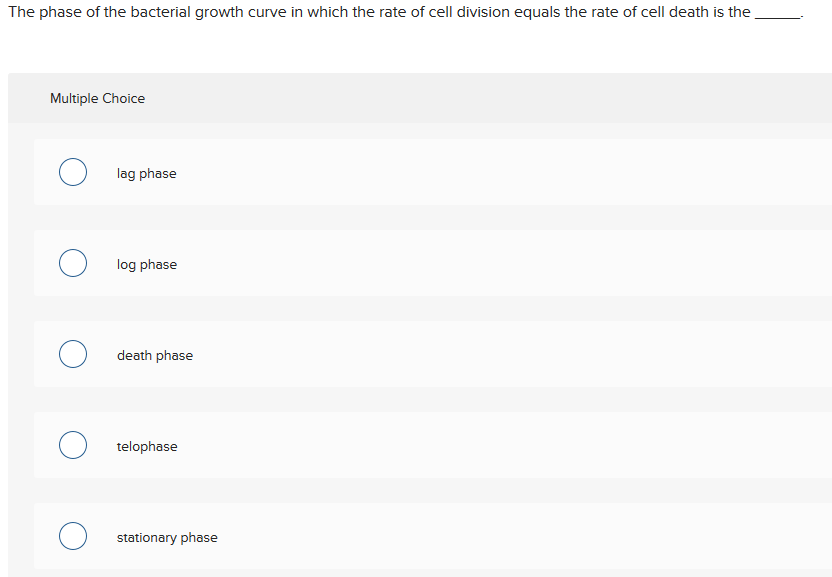A multiple-choice question from a biology-related content is presented on this page. The question reads: "The phase of the bacterial growth curve in which the rate of cell division equals the rate of cell death is the". The provided answer options are:
1. Lag Phase
2. Log Phase
3. Death Phase
4. Telophase
5. Stationary Phase

Despite some uncertainty and lack of background in biology, the respondent deduces that the correct answer is likely the "Stationary Phase", reasoning that other options such as "Death Phase" and "Telophase" seem less likely in this context.